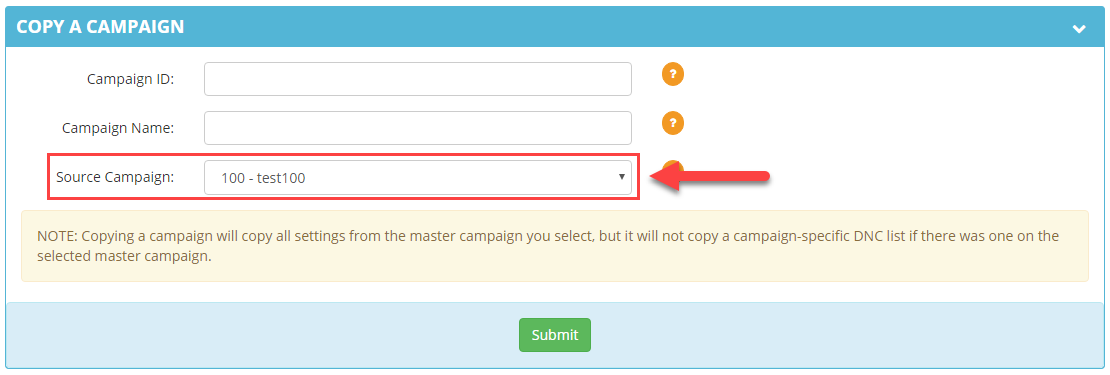The image displays a light blue header at the top with white capital letters reading "COPY A CAMPAIGN." On the right side of the header, there is a downward-pointing arrow icon that presumably opens a dropdown menu when clicked. 

Beneath the header is a white background, where various form elements are aligned. On the left, the first label reads "Campaign ID," next to which is a text box. Adjacent to the text box is an orange circle with a question mark inside, indicating that it might offer additional information upon interaction. 

The next section is labeled "Campaign Name," featuring another text box with a similar orange question mark icon beside it.

Following this, the label "Source Campaign" is displayed, accompanied by a dropdown menu that currently shows the option "100-TEST100." This section is highlighted with a red rectangular box and a red arrow pointing at it from the right side, drawing attention to it.

Below this, a pink rectangular box contains an important note: "COPY A CAMPAIGN OR COPY ALL SETTINGS FROM THE MASTER CAMPAIGN YOU SELECT BUT WILL NOT COPY A CAMPAIGN SPECIFIC DNC LIST IF THERE WAS ONE ON THE SELECTED MASTER CAMPAIGN."

At the bottom of the image, there is a noticeable green button.